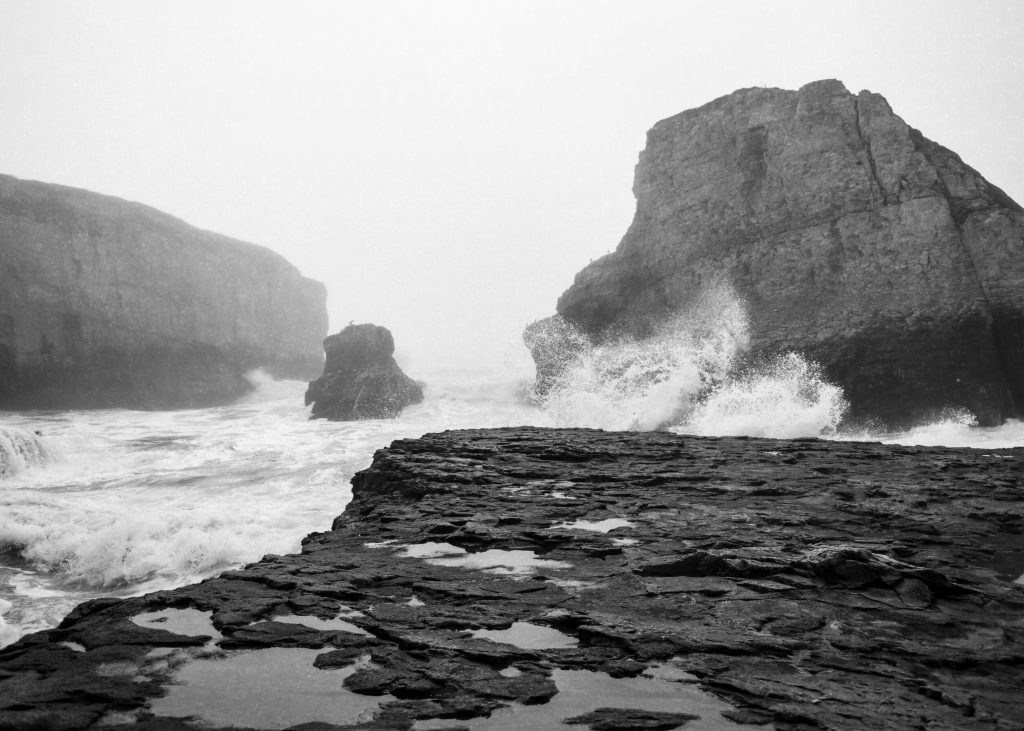This black-and-white photograph captures a dramatic seascape on an overcast day. The scene is framed from a rough, flat rocky plateau overlooking a turbulent ocean. Waves crash violently against various rock formations, creating an intense and dynamic view. In the foreground, the photographer's vantage point is evident from the rocky surface they stand upon. To the left, a steep, tall cliff forms one side of what appears to be a cove or inlet. The right side of the photograph features two larger rock formations, one prominently larger than the other, with waves aggressively battering their bases. The sky above is a uniform gray, shrouded in fog, enhancing the dramatic and moody atmosphere of the coastal landscape. The overall composition emphasizes the powerful interaction between the ocean and the rugged coastline, embodying the raw beauty of nature.